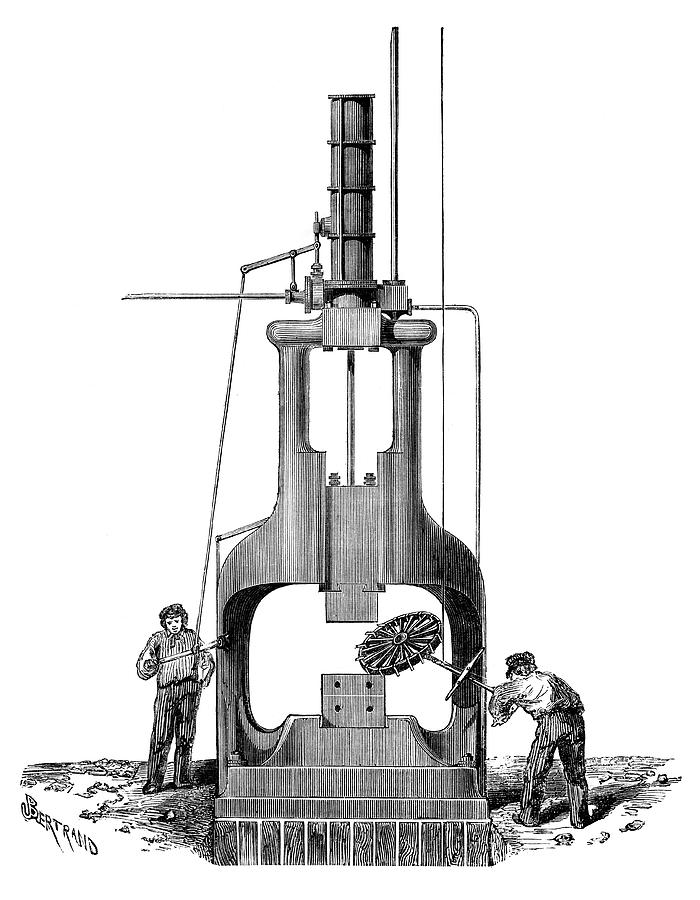The image is a meticulously detailed, black and white drawing featuring a large piece of complex machinery at its center, against a stark white background. The machinery, which resembles a bell with a square base and a narrow cylindrical extension at the top, appears to be the focal point of the workers' activities. The base of the machine is approximately four inches wide, and the entire structure reaches a height of about five inches.

Two workers flank the machine, with one on the left and the other on the right. The worker on the left is seen adjusting a horizontal bar that extends from the base of the machinery, holding it with his right hand. This bar is connected to a string that runs up to a lever at the top, suggesting the worker might be preparing the machine for operation or maintenance. Meanwhile, the worker on the right is using a stick, holding it with both hands to maneuver a small gear or cog located toward the center of the machine, in a gap between two pillars. This gear appears to be part of the intricate workings of the machine, possibly involved in its operational mechanism.

The background is entirely white, emphasizing the detailed line work of the machinery and the workers. In the lower left corner, the name "BERTRAND" is inscribed, possibly indicating the artist or the name of the machinery. The overall impression is that of a highly technical, mechanical apparatus being either assembled or maintained by the two diligent workers.